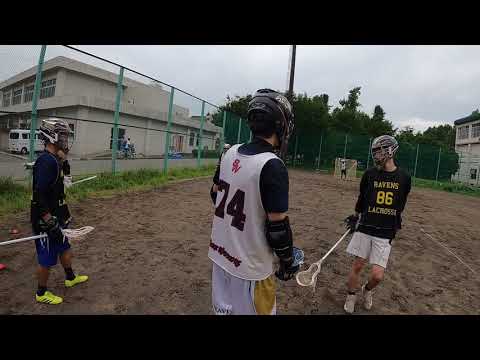The image captures a scene of three high school boys playing lacrosse on a mostly brown dirt field, possibly within a city park, as indicated by the surrounding chain-link fence and nearby buildings. The foreground features three boys standing side by side, each dressed in varied lacrosse uniforms. The boy on the left wears a black jersey, the one in the middle sports a white jersey with the number 74, and the boy on the right is clad in another black jersey emblazoned with "Ravens Lacrosse 86" in yellow font. All three are equipped with helmets and protective gear, holding white lacrosse sticks. In the distant background, a goalie in full gear stands watch in front of his net. The field is enclosed by a green chain-link fence, beyond which are two-story buildings, a white van, and dark green trees under a cloudy, overcast sky. The setting appears somewhat makeshift as the play area lacks grass, suggesting a potentially less-than-ideal playing surface.